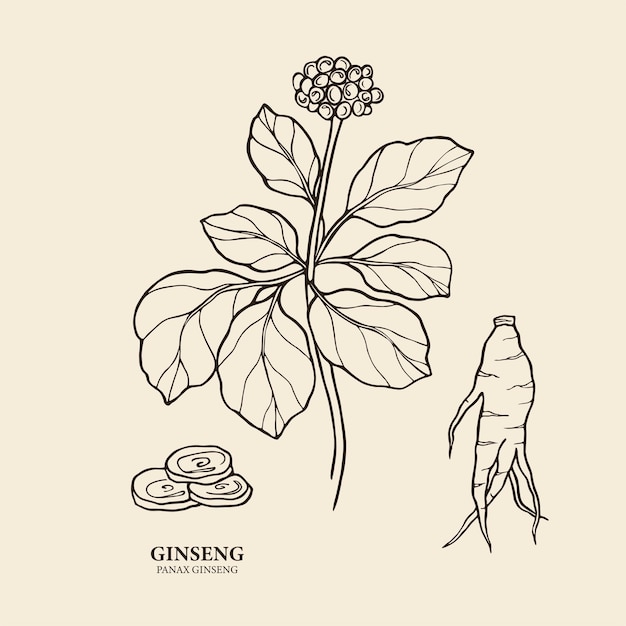This illustration features a detailed, black line drawing on an ivory background. In the lower left corner, the image is labeled in black font with the text "ginseng, Panax ginseng." The drawing prominently includes various parts of the ginseng plant: the central piece is the ginseng root, characterized by its branching, spindly appendages resembling fingers. To the side, we see the plant itself, complete with large, oval, teardrop-shaped leaves and flower clusters that resemble dandelions, each formed from small circles. The illustration also depicts three thin, lateral slices of the root, casually stacked together like a pyramid or a pile of coins. The background of the image has a light tan or beige hue, giving the appearance of a colored paper or photoshopped layer.